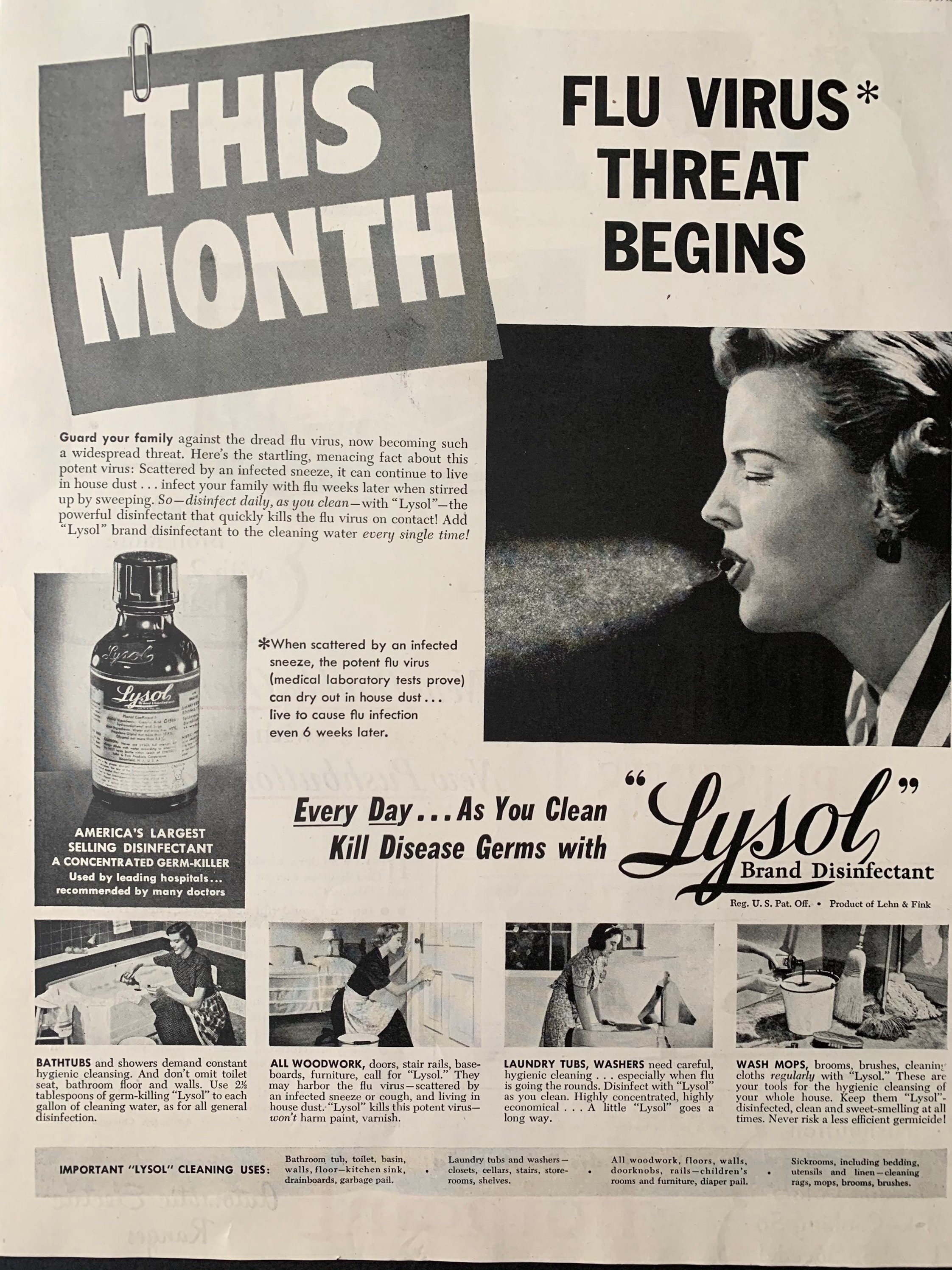This image is a vintage magazine advertisement for Lysol disinfectant, displayed on an off-white vertical rectangular page. At the top, a large gray box with bold white capital letters announces "This Month," while to the right, in smaller black capital letters, the text reads, "Flu Virus Threat Begins." Below this header, there's a striking black-and-white photograph of a woman with curly hair, caught mid-sneeze, with visible particles spewing from her mouth, symbolizing the spread of the flu virus.

To the left of the woman, a detailed paragraph warns readers about the flu virus, explaining that it can linger in house dust and reinfect family members weeks later. The text urges daily disinfection using Lysol, emphasizing its potency in killing the flu virus on contact by adding it to cleaning water.

Beneath this explanatory text, a prominent image of a Lysol bottle is featured, labeled as "America's Largest Selling Disinfectant" and described as a "concentrated germ killer." To the right, more bold text reiterates the key message: "Every Day as You Clean, Kill Disease Germs with Lysol."

At the bottom of the ad, there are four smaller horizontal images showing a woman cleaning various parts of her home, including a bathtub, a door, a laundry setup, and a scene where she pours Lysol into a bucket. These visuals illustrate the versatile uses of Lysol in everyday cleaning, reinforcing the ad's central theme of protecting the home from disease germs.